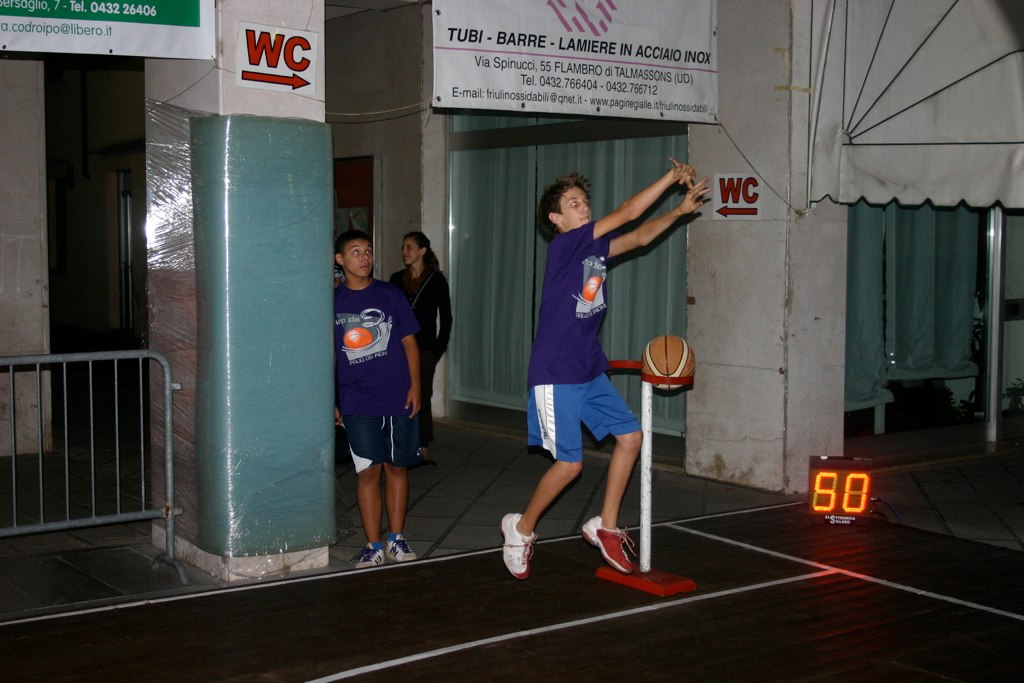In this image, we observe a sporting event, possibly a free throw contest, taking place in a gymnasium. The scene focuses on a young male, appearing to be in his early to mid-teens, who has just thrown a ball. He wears a purple shirt with a graphic depicting a basketball hoop, blue shorts, and distinctive white and red sneakers. His arms are extended in front of him, suggesting the motion of shooting a basketball. Beside him stands a white and red stand holding another basketball at waist height, ready for use. 

A digital timer on the floor next to the stand displays the number 50 in large orange digits. Behind the boy, another male, also in a purple shirt, leans against a pillar, observing the action. Both individuals are part of the same team, indicated by their matching jerseys. In the distant background, a woman smiles while looking off to the side, adding a touch of warmth to the scene.

The gymnasium is equipped with pillars, posts, and barricades, with striped flooring visible in the foreground. A prominently placed banner above the young athlete is inscribed in Italian, reading "TUBIBARRELAMIEREREINACCIAIOINOX." Further clues to the Italian setting include a partially legible Italian email address ending in ".it" and a detailed address containing "VIA SPINUCCI 55." Additionally, signage marked "WC" directs towards restroom facilities. The comprehensive details and vivid depiction create a lively snapshot of this competitive and energetic sports moment.